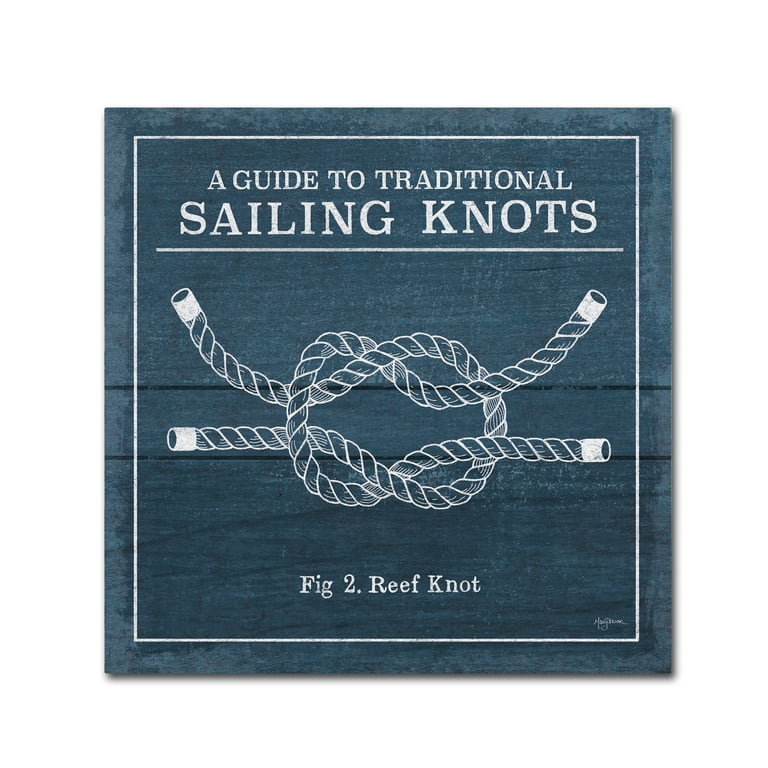The image depicts a square sign designed to resemble a wooden plaque painted in blue with a prominent white square border. At the top of the sign, white uppercase text reads "A Guide to Traditional Sailing Knots." Below this title, the sign features a detailed diagram of a reef knot, labeled as "Figure 2: Reef Knot." This knot, formed by two white rope ends twisted together, resembles a pretzel shape. The background of the image is solid white, accentuating the blue and white colors of the sign, giving it a nautical and rustic aesthetic that suggests it is part of a handmade guide to traditional sailor knots.